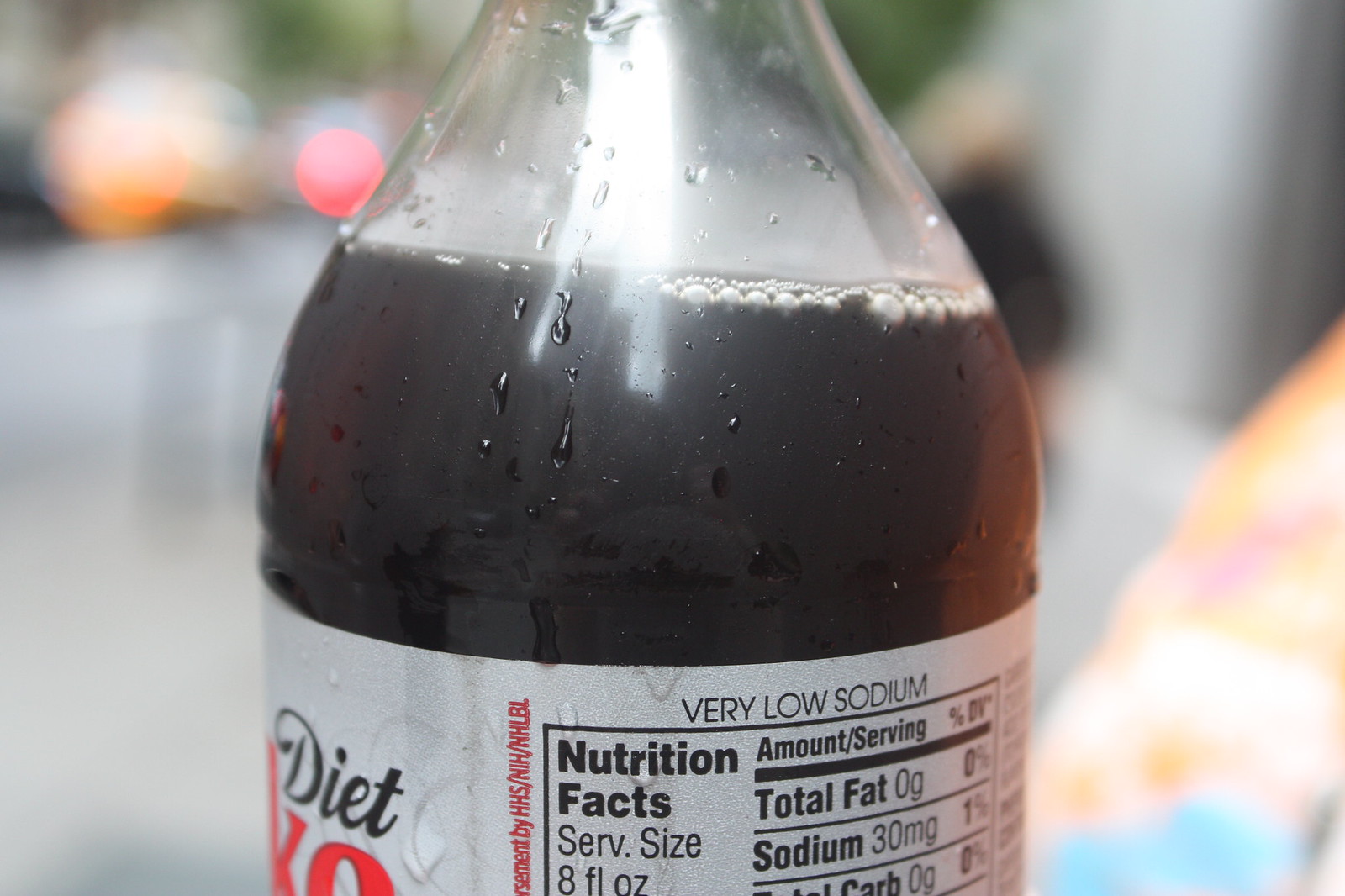The image captures a close-up of a Diet Coke bottle with a slightly blurred background. The photograph focuses on the upper portion of the bottle, starting from midway up to just below the cap. The bottle contains dark brown liquid with a few bubbles at the top, indicating it has been opened and a small amount consumed. The bottle’s label is light gray, featuring the word "Diet" in black letters and "Coke" in red. Both the nutrition facts and other label details are prominently visible on the right side, listing information such as an 8 fluid ounce serving size and the notice "very low sodium." The backdrop hints at an outdoor setting, showing lights on the left side and a sidewalk or road. Additional background elements include a colorful item with shades of orange, white, pink, and blue in the bottom right corner, as well as a person standing in the top right section, all adding layers of context to the scene.